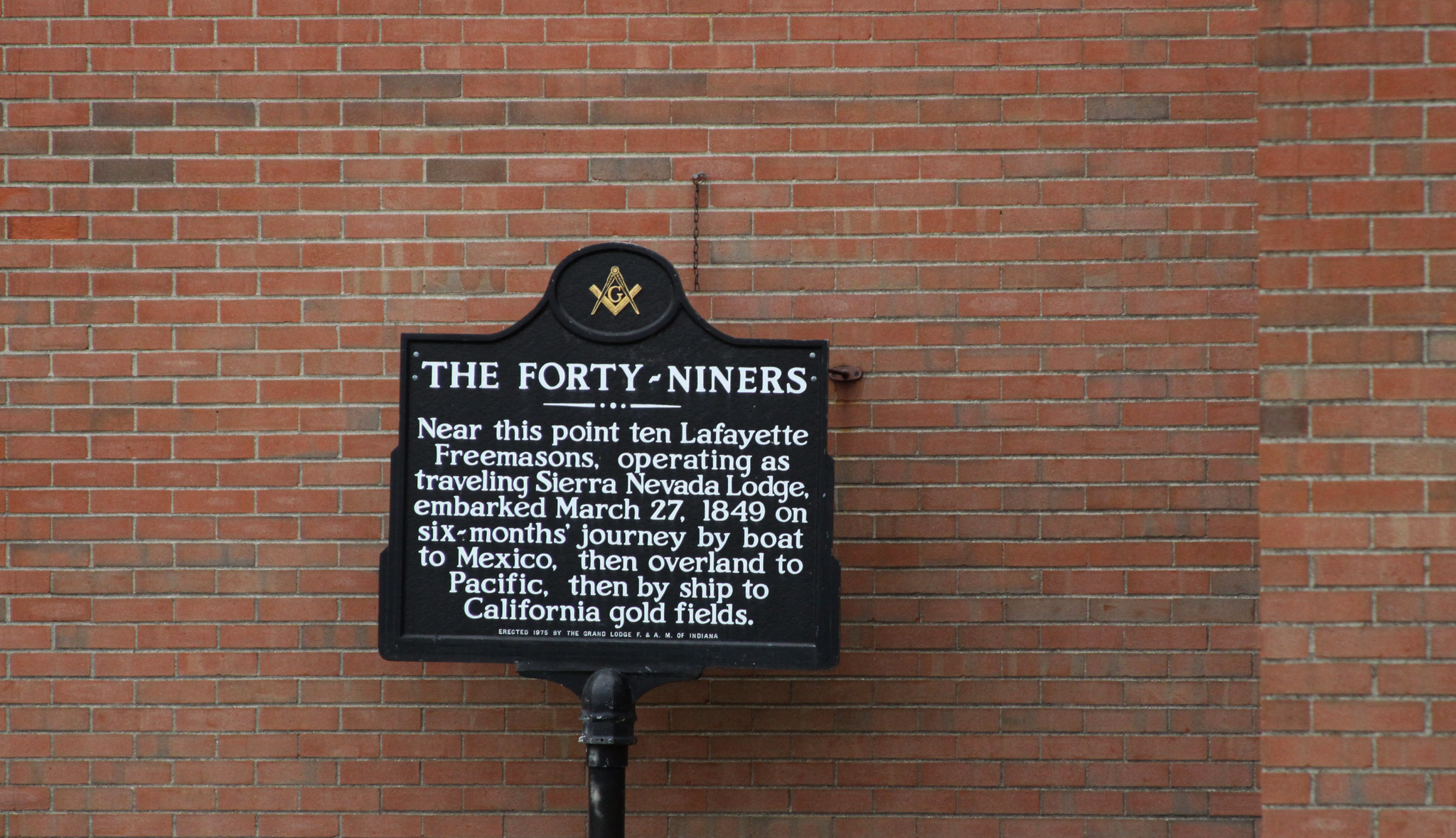The image showcases a historical marker against a predominantly red brick wall, interspersed with some gray bricks. The marker is a black sign with white text and features a gold emblem at the top—a gold 'G' flanked by an upside-down 'V' and a regular 'V'. The sign reads: "The 49ers" in bold, followed by an inscription detailing a significant event. It recounts how ten Lafayette Freemasons, part of the Traveling Sierra Nevada Lodge, embarked from this point on March 27, 1849, on a six-month journey by boat to Mexico, traveled overland to the Pacific, and then continued by ship to the California Goldfields. This marks an important moment in history, akin to modern-day pioneering ventures. The sign is supported by a black stick and leans slightly against the textured brick wall.